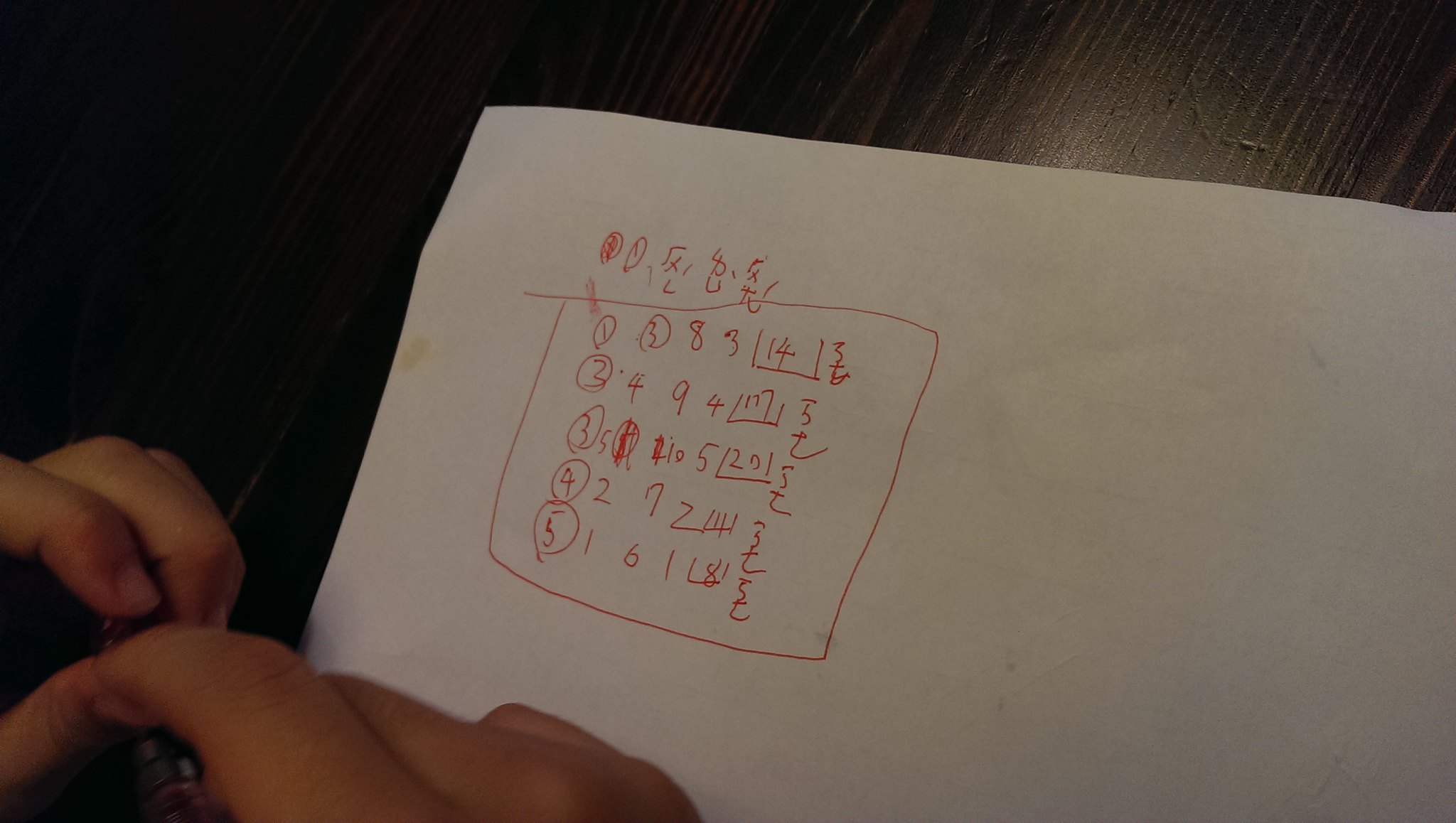A detailed photo caption could be:

On a dark brown wooden table, with clearly visible wood grain lines, lies a piece of paper. A person's hands, possibly male and of fair complexion, hover slightly above it, holding an object resembling a vape. The person appears to be using an unusual-looking red pen to write or draw on the paper. The paper itself features a large, hand-drawn square alongside a series of intricate markings. Above the square, there are a few numbers encircled, as well as some X's and 8's. Within the square, a sequence of numbers from 1 to 5 are each circled and listed vertically. To the right of each circled number is a set of three numbers, followed by a half-square with an open top containing additional numbers. Further right, there appears to be a fraction or possibly a symbol written beneath another number.